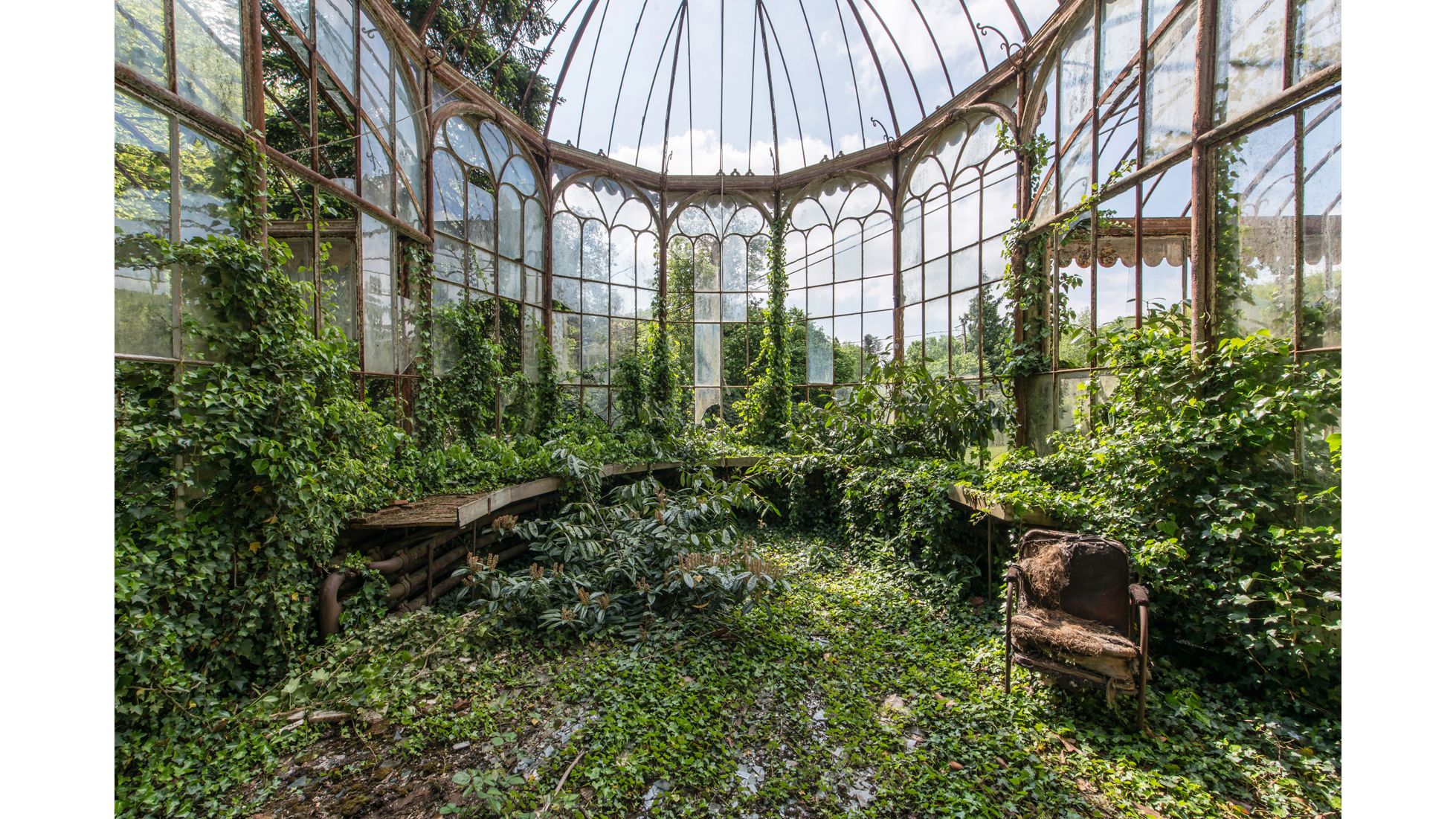The photo depicts a vintage English greenhouse with a distinct oval or domed shape, framed entirely in iron or metal. The structure features decorative arched and square glass panels, many of which are missing, particularly from the roof. Inside, the greenhouse is overrun with English ivy and various other foliage, suggesting a once-cultivated space now reclaimed by nature. The ground is lush with greenery, and the walls are densely covered in ivy, demonstrating a significant overgrowth. Among the remnants of human touch, there is a ratty, torn outdoor chair on the right side and wooden slats or benches partially submerged under the vegetation. The scene is bathed in bright sunlight, with a backdrop of light blue skies and white clouds visible through the remaining glass panels. The overall impression is of an abandoned, once-grand structure now blending seamlessly into the encompassing garden, possibly part of an old estate or castle grounds.